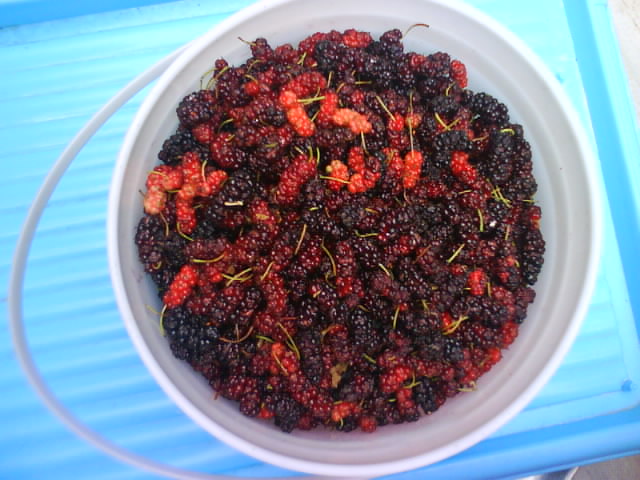In this overhead photographic shot, a white plastic bucket, placed on the glass ledge of a refrigerator and backlit to a blue hue, is filled to the brim with an assortment of raspberries and blackberries. The berries, varying in color from light red to dark black, still have many tiny green stems attached, adding a touch of green accent amid the dense field of red and black. The bucket's handle rests on the left side in a down or side-to-waist position. The bright, reflective blue light from below enhances the image, drawing attention to the texture and organic quality of the berries, suggesting they are freshly picked and natural. The viewer's perspective is limited to the interior contents and the rim of the bucket, with no exterior or people visible in the shot.